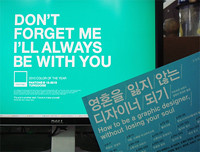The image depicts a low-resolution (approximately 256 pixels) computer monitor with a black border and a white base. The screen displays a light teal background with the message, "Don't forget me, I'll always be with you," written in large white letters at the top, followed by additional white text below. Positioned diagonally in front of the monitor’s lower right corner is a blue card containing both Korean characters and their translation, which reads, "How to be a graphic designer without losing your soul." The card partially obscures the bottom of the monitor, making the monitor’s brace and some background details slightly visible but indistinct. The scene appears to be indoors, possibly in a lobby setting.